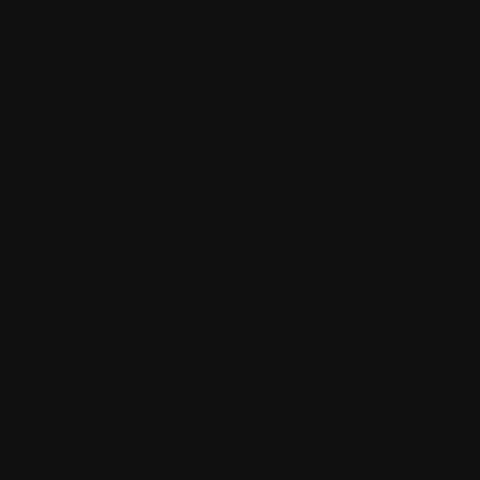A completely solid black square with no discernible features. The image contains no objects, text, or variations in shading or texture. It is a uniform black square devoid of lines, shadows, or any other elements. The stark simplicity and unchanging nature of the black color may give an illusionary sense of depth or glow upon prolonged viewing, but it remains unmarked and featureless.